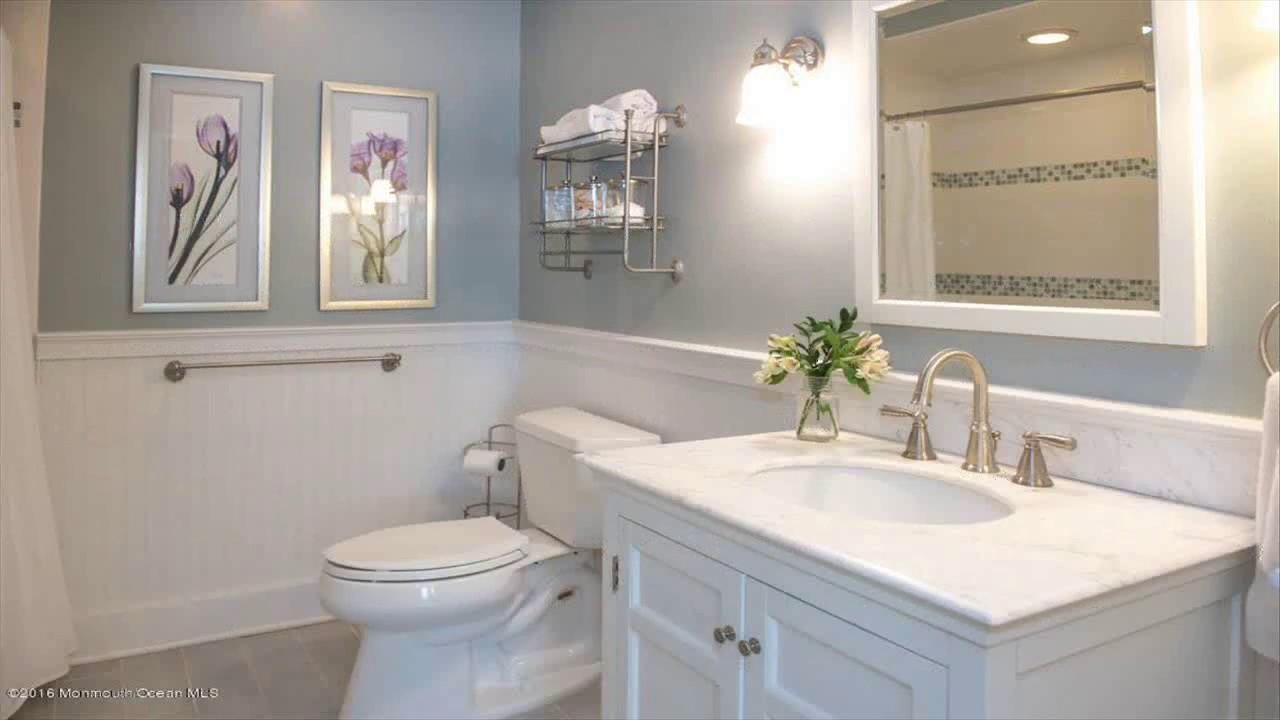The photograph captures a meticulously designed bathroom interior. The lower half of the walls is adorned with white wainscoting, featuring vertical wooden slats and complemented by a white baseboard and trim. In contrast, the upper walls are painted with a matte gray hue, creating a sophisticated dual-tone effect. The bathroom fixtures, all finished in a sleek silver, exude a modern elegance.

A single sink serves as the room's focal point, boasting a gracefully curved faucet flanked by two handles. The countertop and backsplash are crafted from pristine white marble, enhancing the space's luxurious feel. Below the counter, the sink is set into a cabinetry unit with double doors, painted in a classic white.

To the right of the sink stands a clean, white toilet. A toilet paper stand is conveniently placed in the corner next to it. Adjacent to the toilet, a towel bar remains unadorned for now, situated beneath two pieces of framed artwork. Each piece features a floral motif on a white background, bordered by gray and framed in silver and light brass, respectively.

Mounted above the toilet is a rack, neatly stocked with folded towels and assorted toiletries. A wall-mounted light fixture casts a warm, downward glow, while directly behind the sink, a large mirror with a white square border reflects the room’s details, adding depth and brightness to the space.